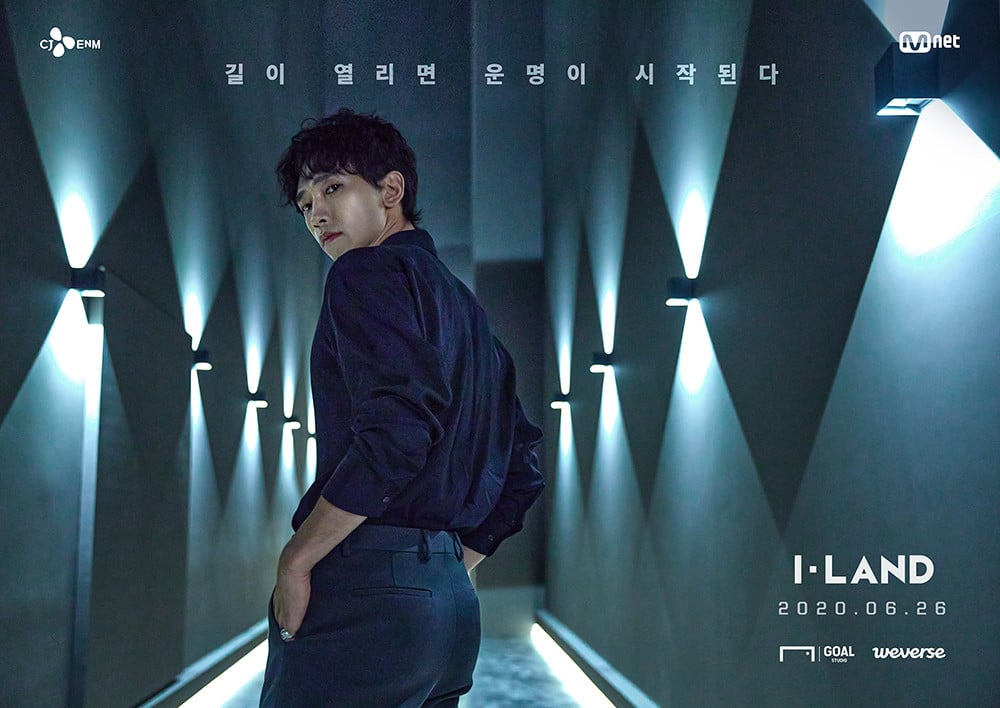In a dimly lit corridor, an Asian-American man stands with his back partially turned, glancing over his shoulder. His hands rest in the pockets of his dark pants, one of which displays a ring on his little finger. The man, appearing to be in his early twenties, wears a black shirt, and his black hair is combed down to his ears. The corridor, characterized by its dark green walls and concrete floor, is illuminated by a series of turquoise lights arranged in a triangular pattern along both sides. There is a solid wall of dark green material at the end of the hallway. Additionally, the image serves as an advertisement, featuring text in Korean at the top and "I land 2020-06-26 goal weavers" at the bottom right corner, with "Mnet" marking the top right corner. His serious expression and the unique lighting add an enigmatic atmosphere to the scene.